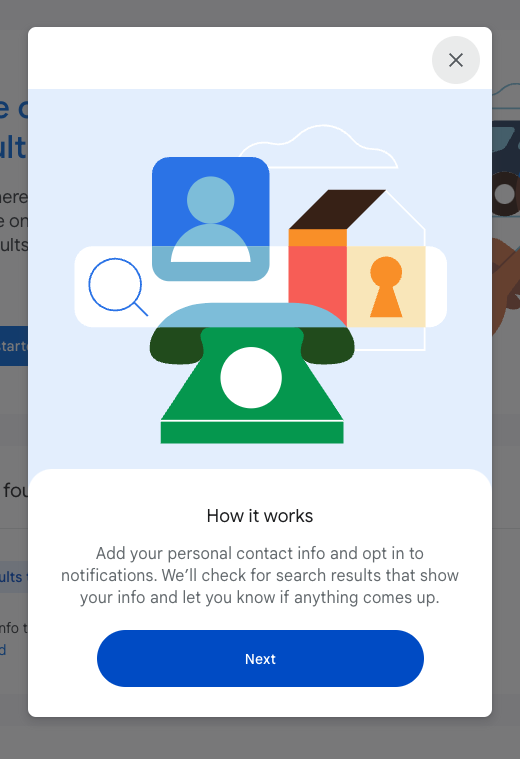The screenshot depicts a notification primarily characterized by Google's design aesthetics. Dominating the upper section is a graphic illustration; it shows a person icon on the left, represented within a blue square. Adjacent to it is an image of a house featuring a yellow lock symbol, indicative of security, and a brown roof. Below this illustration is an icon of a green telephone with its receiver placed down, surrounded by a white circle. 

Underneath this visual, the text header "How it Works" is prominently displayed in black. The accompanying description reads: "Add your personal contact info and opt-in to notifications. We'll check for search results that show your info and let you know if anything comes up." This message suggests that the notification is a prompt for users to enter their personal contact details and agree to receive notifications. This feature appears designed to monitor search results and alert users if their information appears online.

The context of this notification implies its presentation during scenarios such as the initial account setup, logging in on an unfamiliar device, or navigating to the settings page for the first time. The purpose is clearly geared towards enhancing security and managing personal information efficiently.